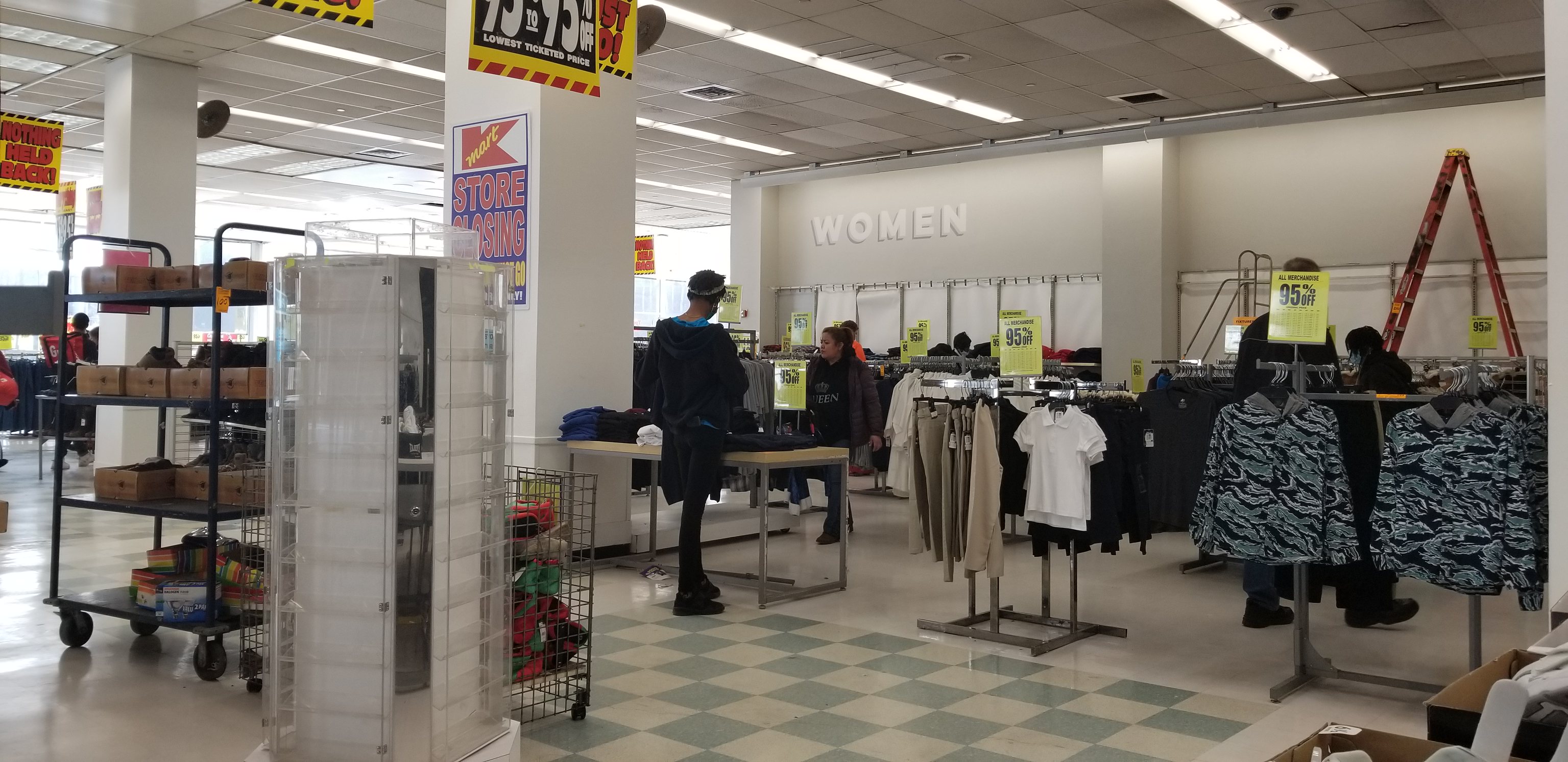This image captures the interior of a Kmart store during a closing sale, characterized by large discounts and a bustling atmosphere. Visible are the iconic red Kmart symbol with yellow writing and several signs advertising markdowns ranging from 50% to an astounding 95% off. The store features light gray walls, including a prominent section labeled "Women" in white text. Adjacent to this is a white column and an array of yellow and red sale signs.

The ceiling, adorned with vents and white panel tiles, casts light onto a checkered green and white floor, which contrasts with another section of white flooring. Centered in the frame is a brown table with silver legs, flanked by numerous racks and carts displaying various clothing items like pants, shirts, and skirts. Notably, a wheeled metal rack with shoe boxes and a wire crate filled with merchandise can be seen.

Shoppers are actively browsing through the discounted items. A girl dressed entirely in black with a black jacket is inspecting a rack, while a gentleman, also in black attire, including a hat, examines goods on a display table. Both shoppers contribute to the scene's sense of activity. In the background, a red ladder stands out against the shelves, which house boxed items. In the upper left-hand corner, more people are seen perusing the clothing on offer, reinforcing the store's busy atmosphere during this significant sale event.